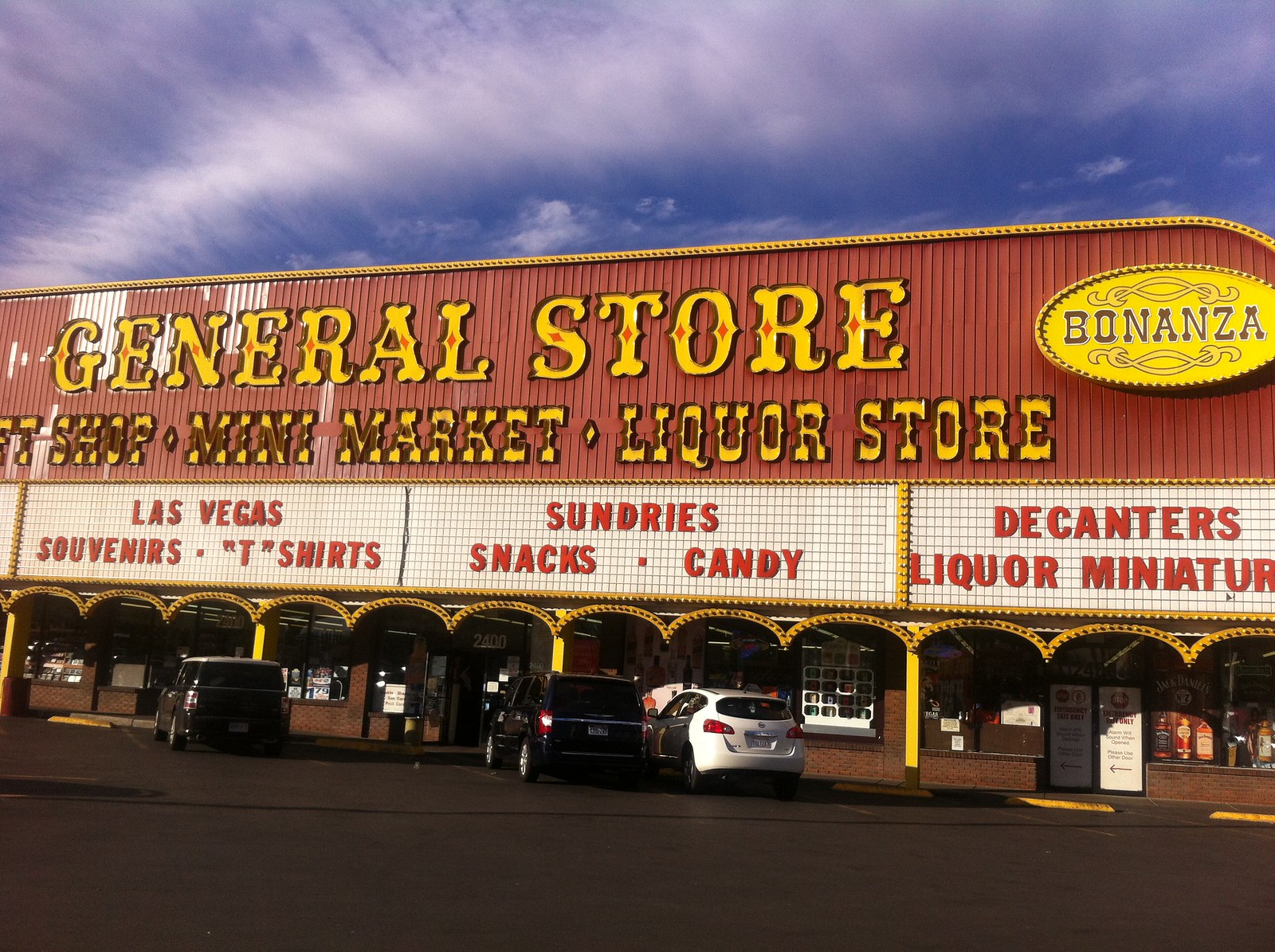The image shows the exterior of a large brick store under a blue, partly cloudy sky. The top part of the building's facade is red, prominently displaying "General Store" in large yellow letters. Adjacent to this, a circular sign reads "Bonanza." Below, in smaller text, the sign states "Mini Market Liquor Store," with additional descriptions mentioning "gift shop." Continuing downward, a white marquee with red typography lists various items such as "Las Vegas souvenirs, t-shirts, sundries, snacks, candies, decanters, and liquor miniatures."

The store's lower facade features small arches supported by yellow poles, leading to visible windows and doors. One door is marked with the number "2400." The parking lot in front of the store is occupied by a white car and two black cars, all facing slightly left. The overall scene is framed by the blue sky above, speckled with clouds, suggesting a pleasant yet possibly stormy day.